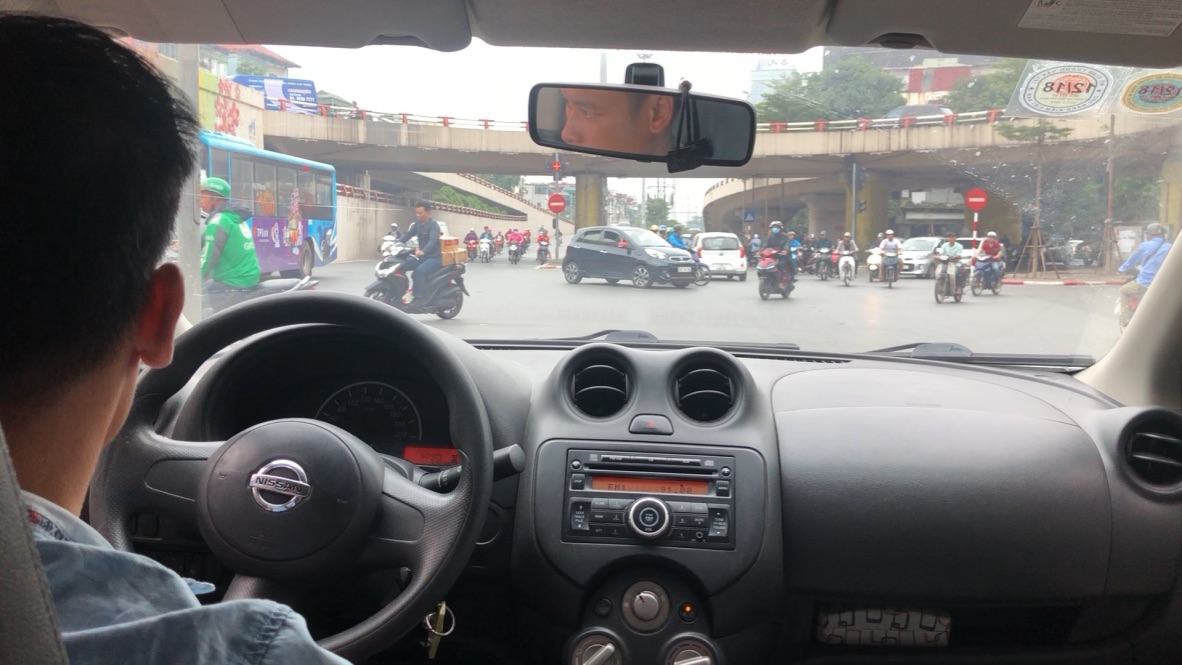This detailed color photograph captures the interior of a Nissan car from the vantage point of the middle of the back seat. The dashboard and steering wheel, which are predominantly gray, dominate the left side of the image. The Nissan logo is visible in the center of the steering wheel. Just beyond the driver's seat, a partial view of the driver is visible, showing his pale skin, possibly indicating he is either Caucasian or Asian. The driver has dark, crew-cut hair and is wearing a light blue shirt. Through the windshield, a substantial bridge can be seen spanning the road ahead, while several motorcycles are approaching in the opposite lane, adding a dynamic element to the scene.